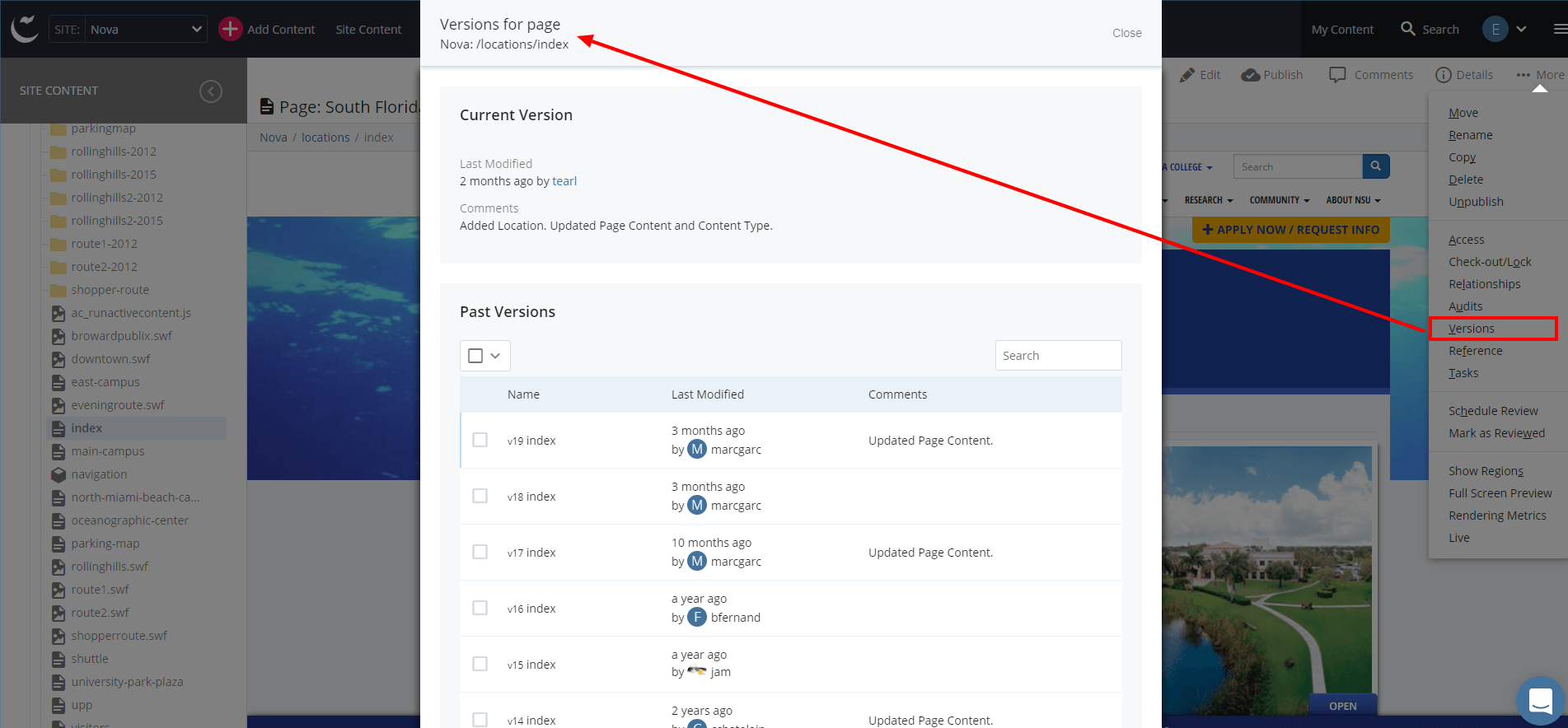This image is a screenshot taken from a laptop displaying an application interface. The text is small and challenging to read, but the screenshot appears to be used for demonstration or training purposes, indicated by a prominent red arrow overlaid on the web page. The web page in focus pertains to South Florida and highlights different versions available for a specific web page. It seems to be an archive or a version control system, showcasing various iterations and content changes made to the website.